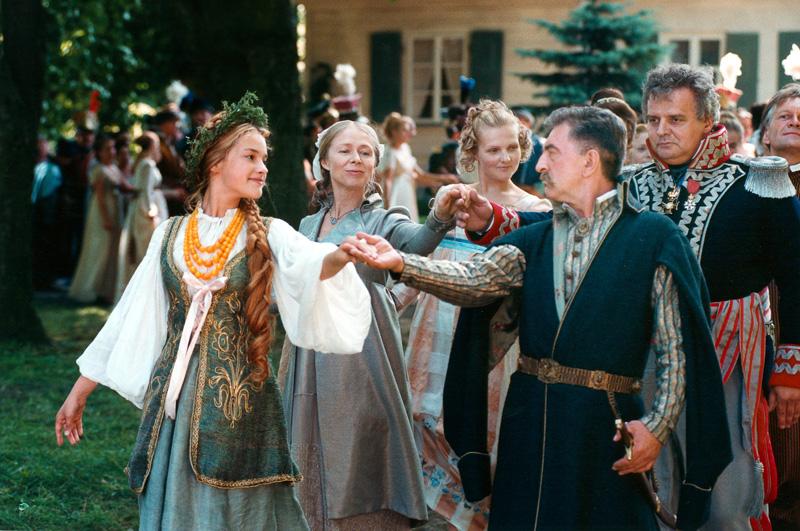In the foreground of this vibrant medieval-themed photo, a young woman with long, dark blonde hair braided over her shoulder, adorned with a green leaf crown, smiles warmly. She is elegantly dressed in a white, flowy shirt with big, open sleeves, and a green and gold embroidered vest, complemented by a large yellow beaded necklace and a green skirt. Holding her hand is an older man with grayish-brown hair and a gray mustache, donning a button-down long-sleeve shirt beneath a green and gold cloak, and clutching a sword in his other hand. Behind them, several other participants, including an older woman and another young lady, also hand-in-hand, join the procession. This scene, set on vibrant grass with a pine tree and a large brown building in the background, captures the essence of a medieval dance pageant or possibly a father-daughter cotillion, evoking the charm and elegance of King Arthur's days.